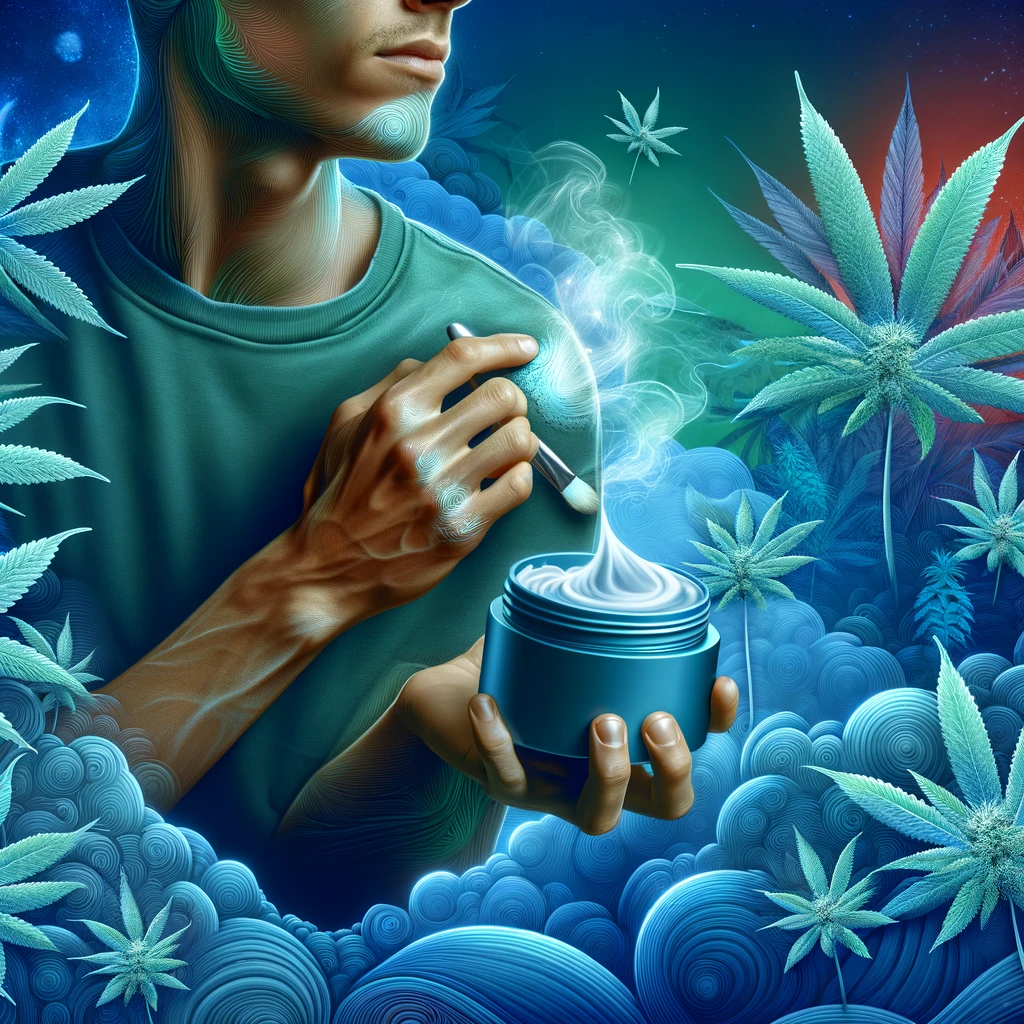In the detailed drawing, only the lower half of a white male's face is visible, extending from his nostrils to his shoulders. He is dressed in a green, open-neck shirt. His right hand, which shows prominent veins, is raised and holds a slender brush pointed towards a round tub of cream in his left hand. White, wispy smoke or cream swirls rise from the tub, creating an ethereal effect. Surrounding him is a rich tapestry of elements: green leaves, possibly marijuana, emanate from the lower left and upper right, while dark blue clouds and swirls drift around him. In the top left corner, a blue light resembling a distant moon adds to the mystical atmosphere. Red and orange hues infuse the upper right corner, contrasting with the darkness at the very top. The scene conveys a dreamlike quality, enhanced by a starry sky and various foliage, clouds, and bubbles enveloping the figure.